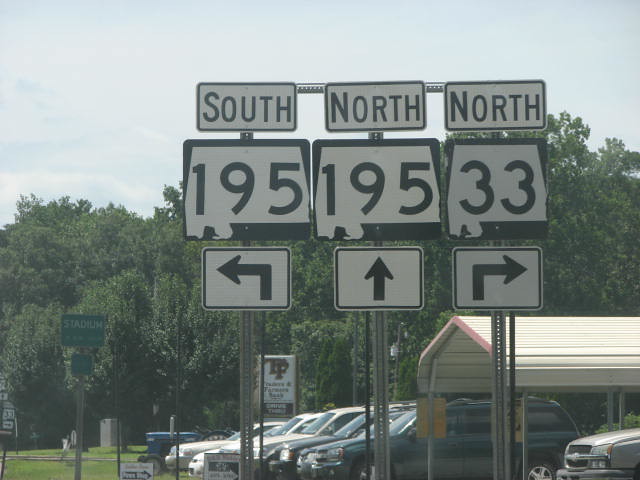The photograph captures a cluster of three signposts situated beside a road, each featuring a set of three signs. On the left post, the top sign reads "South," followed by a weathered "195" sign with a noticeable chip in the lower left corner, and beneath that, an arrow pointing up that then sharply turns left. The center post features "North" at the top, with "195" underneath, and a straight arrow pointing vertically. The post on the right displays "North" at the top, followed by a "33" sign, with an arrow pointing up that then veers to the right. All three signposts strikingly share a peculiar tear in the lower left edge of their signs, almost resembling a duck shape. This tear raises the question of whether the image might be digitally altered. In the background, a parking lot filled with several parked cars can be seen, framed by dense, tall trees. Additionally, a green sign reads "Stadium," suggesting the location might be near a sports facility. Closer to the ground, another sign partially hidden by grass displays the letters "T" and "P" or "T" and "F," possibly alluding to the name of the stadium.